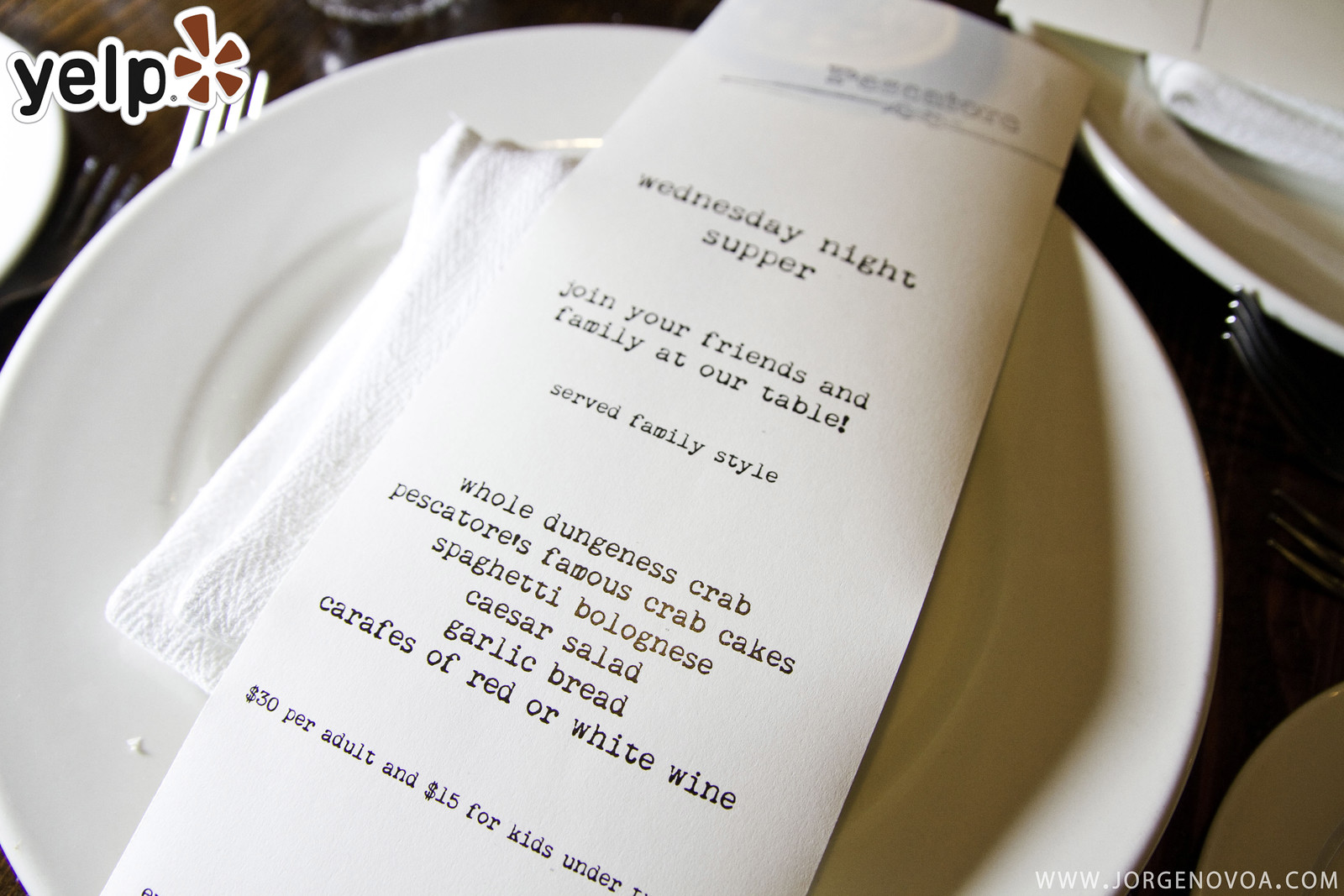The image is a wide rectangular photograph featuring a wooden brown table set for a Wednesday Night Supper. Central to the composition is a white dinner plate, slightly shifted to the left, with a white napkin folded in a V-shape pattern resting on it. On top of the napkin lies a long, rectangular piece of paper resembling a receipt, positioned diagonally from the bottom left corner to the upper right. The receipt details the menu in lowercase black text, listing items such as whole Dungeness crab, spaghetti bolognese, garlic bread, and carafes of red or white wine, priced at $30 per adult and $15 for children. The text encourages diners to join friends and family for a family-style meal. The upper left corner features the Yelp logo, while the bottom right includes the URL www.jorge.navoa.com in white, all-caps. Silverware and additional plates are partially visible to the right, amidst a mildly cluttered table setting.